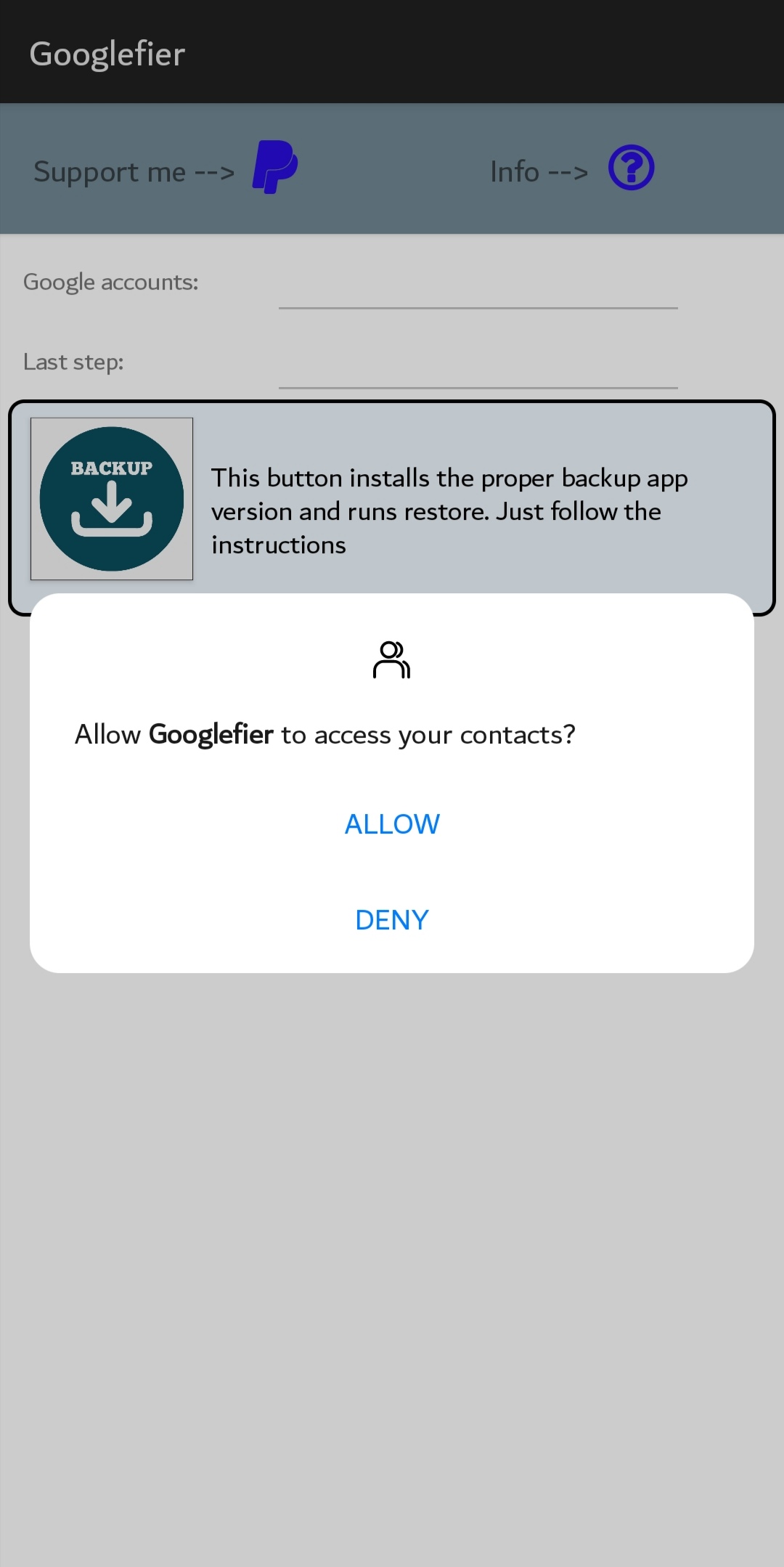**Detailed Caption:**

This image is a screenshot of a mobile application titled "Googlefier," prominently displayed at the top in white letters on a black bar. Directly beneath this title are the words "support me" with an arrow pointing towards a PayPal icon. Adjacent to this, another label "Info" is paired with an arrow leading to a circular icon that contains a question mark. Further down, there is a section labeled "Google accounts" followed by the words "Last step," leading to a central feature within the screenshot: a square containing a black circle. Inside this black circle, "Backup" is written in white letters, accompanied by a downward-pointing white arrow that extends into a curved horizontal line. Below this, an instructional text explains, "This button installs the proper backup app version and runs restore. Just follow the instructions."

Near the bottom of the image, a white pop-up dialog prompts the user with the message: "Allow Googlefier to access your accounts," offering two button options: "Allow" and "Deny." The overall orientation of the image is taller than it is wide, with no photographic elements, people, animals, birds, plants, flowers, trees, buildings, or automobiles present in this screenshot.